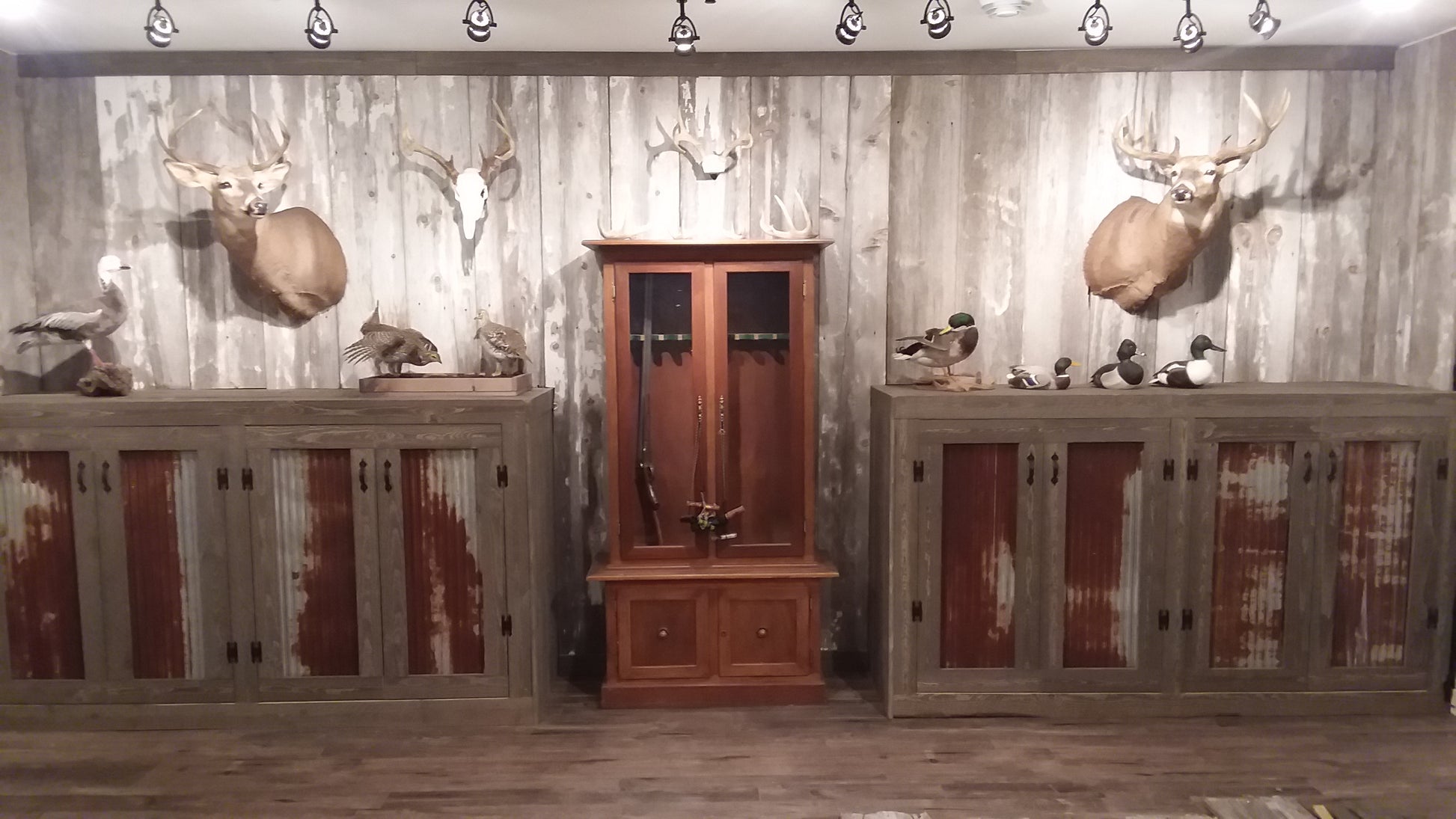The photograph captures a meticulously arranged countryside-themed rustic trophy wall. The back wall, fashioned from light gray planks, serves as a backdrop for an array of hunting trophies. Prominently featured at the center is a brown wooden gun rack with two clear glass windows and two drawers at its base, housing a single rifle. Flanking the gun rack are two clean, light gray wooden cabinets with rustic, rusty sheet metal panels on the doors. Each side of the wall is adorned with a stuffed deer head, positioned at a slight inward angle towards the center of the display. Below the deer heads, smaller mounted taxidermy figures of mallards, ducks, and assorted birds add to the decor. Central to the display, a collection of antlered skulls underscores the theme, completing this snapshot of a carefully curated hunting room.